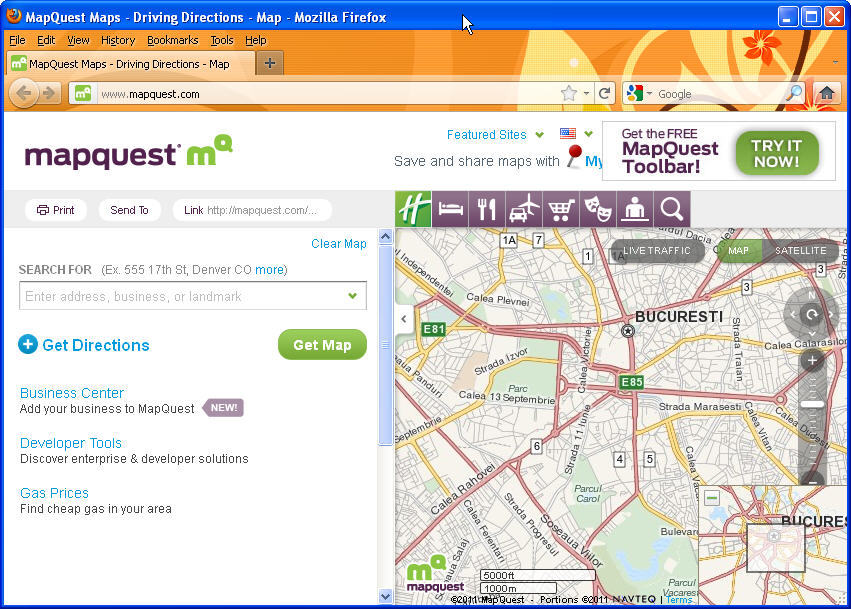Screenshot of a typical Windows dialog box showcasing the Mozilla Firefox browser with the MapQuest website loaded. At the top, a blue bar with a blue outline is visible, featuring the Firefox logo on the far left followed by the text "MapQuest Maps, driving directions, map - Mozilla Firefox". On the top right corner, standard window control icons for minimizing, maximizing, and closing the window are present.

Beneath this top bar is an orange menu bar listing options: File, Edit, View, History, Bookmarks, Tools, and Help. Below the menu bar, a tab labeled "MapQuest Maps, driving directions, map" is open, with a plus sign adjacent for opening new tabs. Immediately under these elements are the browser's navigation buttons (left and right arrows), a search bar displaying the URL "www.mapquest.com", and an additional Google search bar to the right. There's also a small home icon present.

In the main content area of the page, the MapQuest logo is partially visible with "M-A" highlighted in green. The right side of the screen displays a map, while the left side contains a search input example for "555 17th Street, Denver" with options for "Get Directions" and "Get Map" present as interactive buttons.